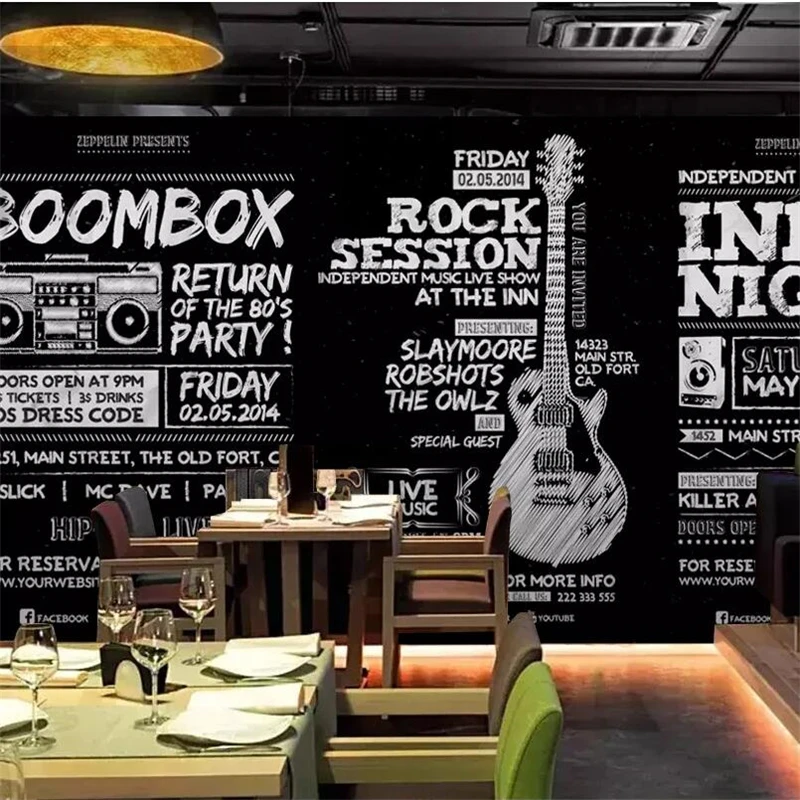The image showcases the interior of a restaurant dining room with an industrial aesthetic, featuring a plain grey concrete floor circled by ambient lighting. Prominently displayed on a black wall is a detailed black and white sign, which reads: "Zeppelin Presents, Boombox, Return of the 80s Party, Doors open at 9pm, Tickets, $50, Drink, Dress Code, Friday, 02.05.2014, 51 Main Street, The Old Fort," and repeats "Friday, 02.05.2014" in the center. Further text promotes a "Rock Session, Independent Music, Live Show at the Inn, Presenting Slaymore, Rob Shots, The Owls, and Special Guest, Live Music." Accompanying the text is a scratched image of a guitar and the phrase "You are Invited, 14.323 Main Street, Old Fort, California." More text indicates phrases such as "Independent" and "Presenting Killer A," although some parts are cut off.

In the bottom left, there are two distinct table settings. One table features a light wooden surface with green place settings, including wine glasses and white napkins, accompanied by wooden chairs with green cushions. The adjacent table in the background is light brown with a setting of white napkins, red and black chairs, and wine glasses. Together, these elements create an inviting atmosphere, ready to host guests, with the black and white decor along the wall further enhancing the ambiance with its nod to rock music and an 80s party theme.